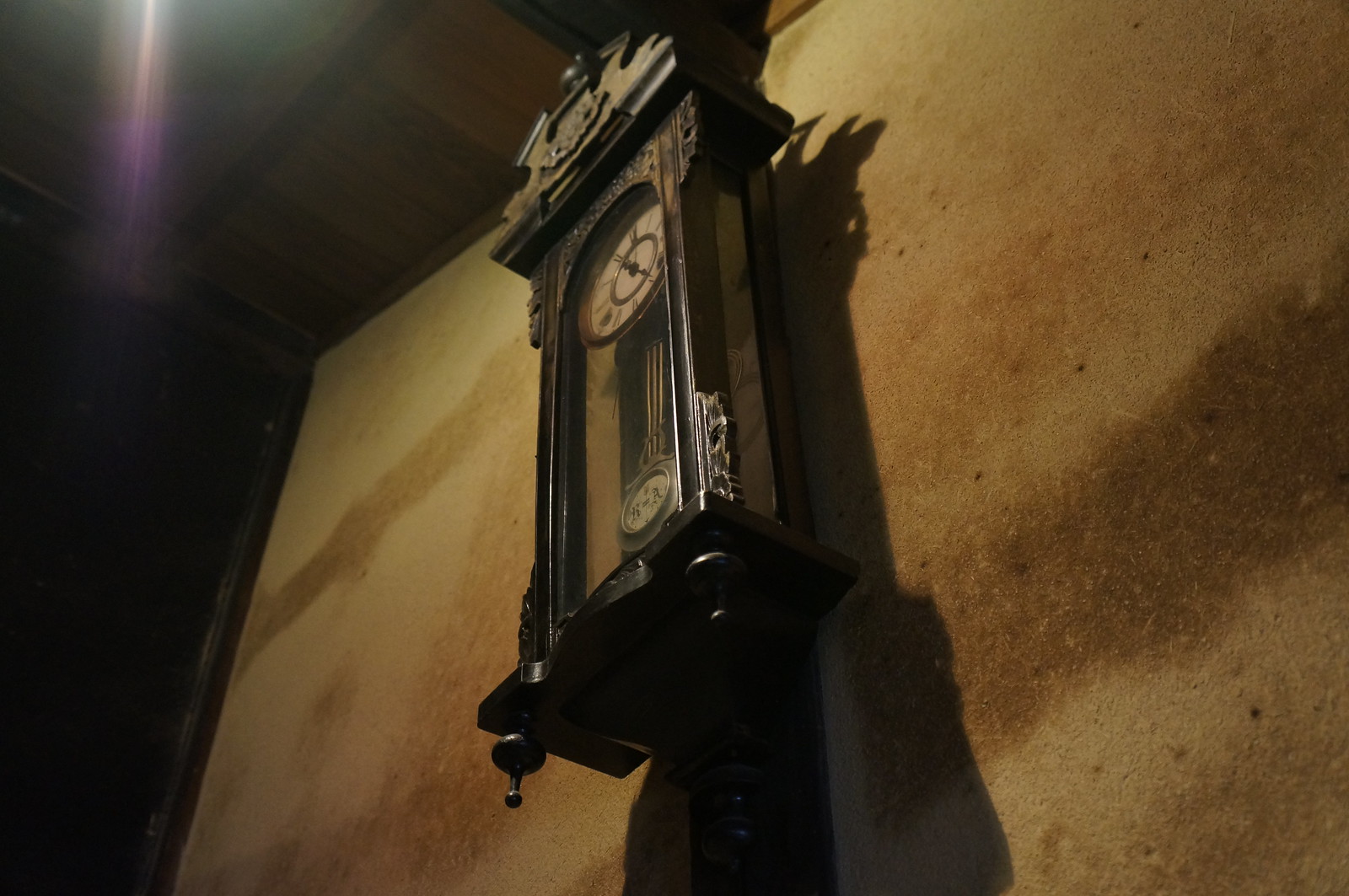A close-up image of an intricately designed stone wall with a prominent antique clock mounted on it. The clock, encased in glass, features a blend of light and dark wood, enhancing its vintage charm. The clock face showcases both numbers and Roman numerals, with a meticulously crafted pendulum swinging below – a slender rod ending in a circular disc at the bottom. The top of the clock boasts ornate decorative carvings, adding to its elegant appearance. Ambient light casts a gentle glow from the top left corner, but shadows cast by the illumination create dark patches, particularly on the left side of the wall. Adding a touch of mystery, several small dots are scattered across the stone surface. A vertical bar runs along the right side, accompanying the clock's framework, with protrusions at the bottom corners, adding to the complexity of this timeless piece.